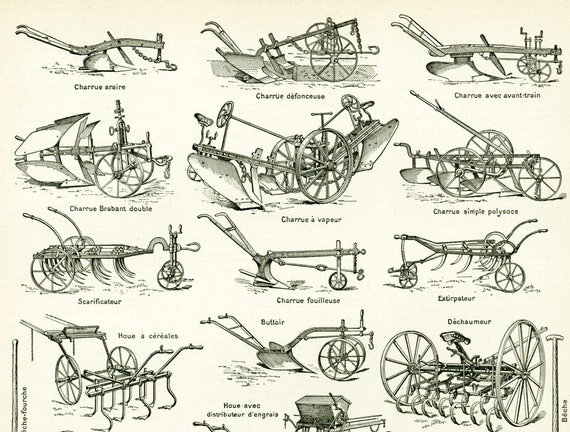The horizontally oriented image is an aged, black-and-white illustration on light beige paper. It appears to be an early 19th-century print showcasing various types of farm equipment, specifically plows and hand implements. The illustration includes around a dozen different tools, each meticulously drawn in black ink. The tools vary in design, with some having one, two, or three wheels, while others are simple harrows without wheels. Each piece of equipment is accompanied by labels and descriptions in French, such as "Charrue" and "Charrue avec avant-terrain," indicating different models and configurations. The equipment appears to be manually operated rather than mechanically powered, suggesting they might have been used with human or animal labor. The layout consists of four rows, each featuring three distinct plows arranged in a realistic and detailed manner, emphasizing the variety and specificity of early agricultural tools.